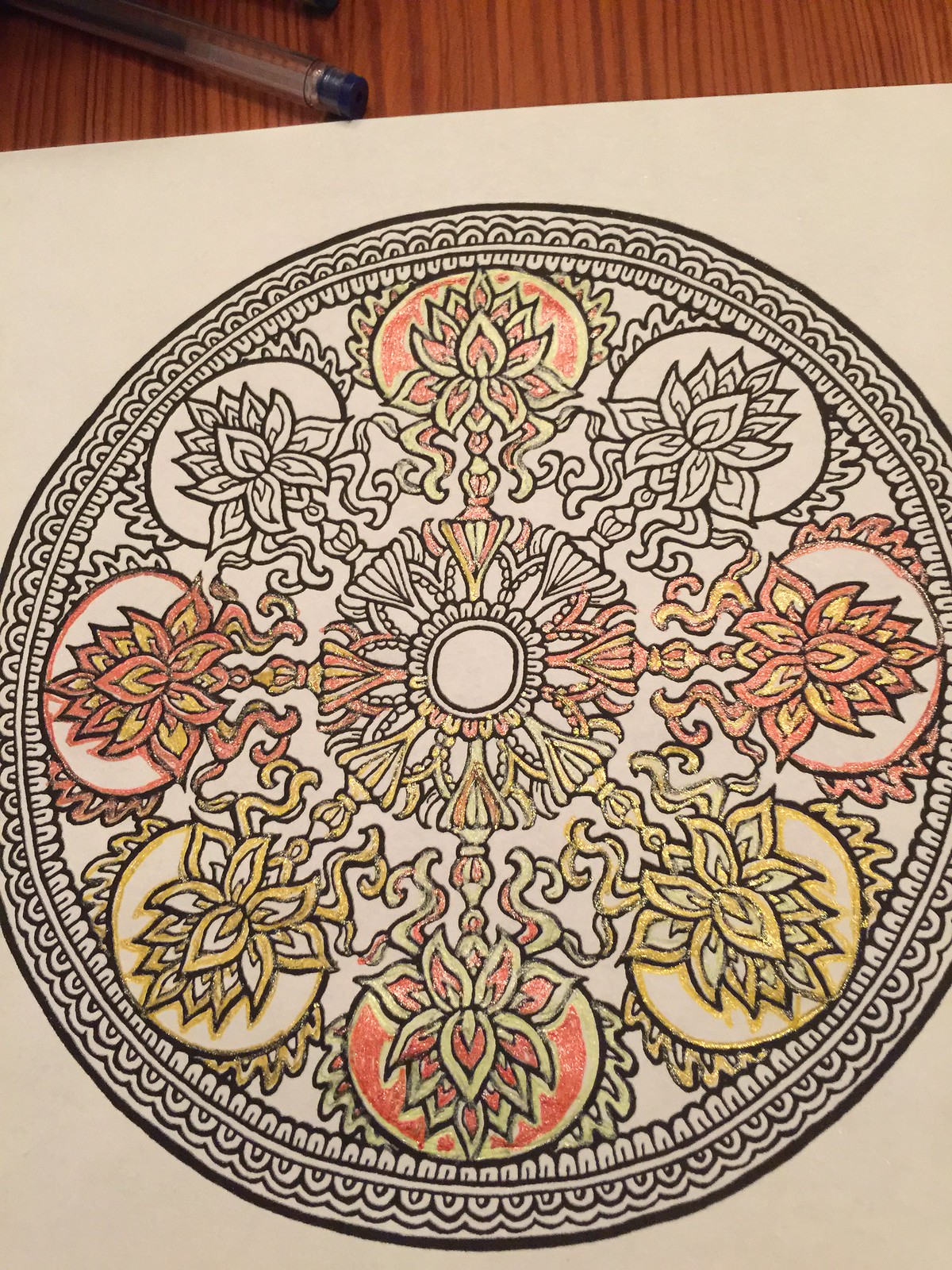This horizontal photograph displays a partially colored mandala coloring page, set against a wood grain surface with a pen visible in the upper left-hand corner. The mandala, outlined in black, is centered within a large circle and features an intricate design themed around a stylized floral motif. At the center is a smaller circle surrounded by small petals, leading out to large, curved thin leaves that terminate in finial-like tops. Beyond these leaves are larger, lotus-like leaves that are wide at the base and thin at the top. The outermost edge is encircled by an oval border adorned with curved lines. Some sections towards the center have been meticulously colored in with rose gold and yellow gold markers, while other petals and leaves incorporate shades of metallic green, red, and orange. The overall design is symmetrical and appears mirrored, with the background left in the natural parchment color of the paper.